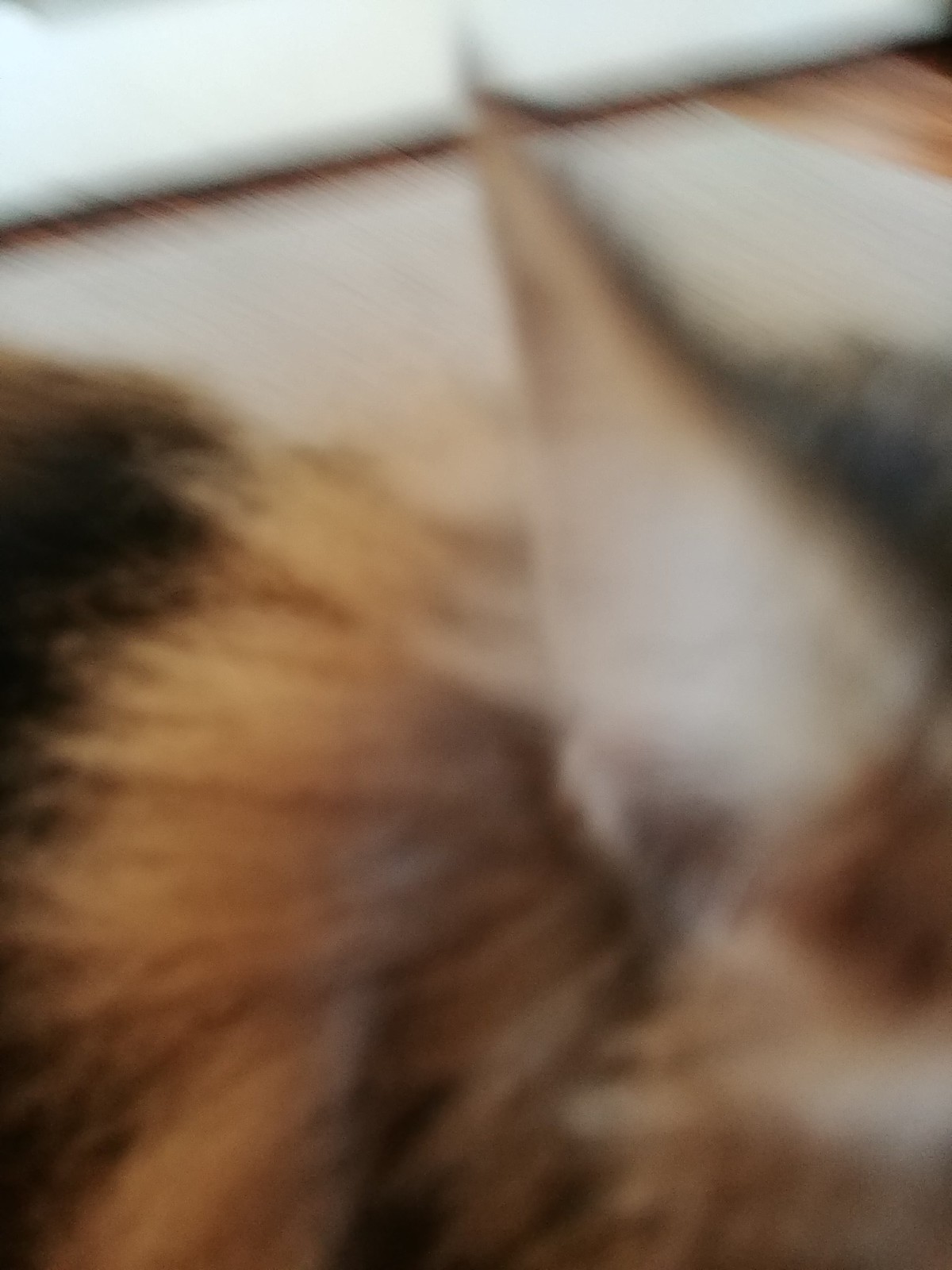This image captures an extremely blurry close-up of a cat's ear, set against the backdrop of what seems to be a living room. The pointed ear, predominantly white on the inside, features long fur that transitions from light brown to dark brown with some white mixed in. The photo suggests the cat was in motion, contributing to the overall blurriness. The setting includes a tan area rug and a brown and white hardwood floor visible in the upper left corner. There appears to be a white couch stretching across the top of the photo, adding to the sense of homely comfort. Though indistinct and smudged, the colors in the image include various shades of cream, brown, and dark brown, with some areas resembling a reddish-brown hue. The cat's face is not visible, as the close-up is tightly focused, featuring two-thirds of the cat’s body stretched from right to left.